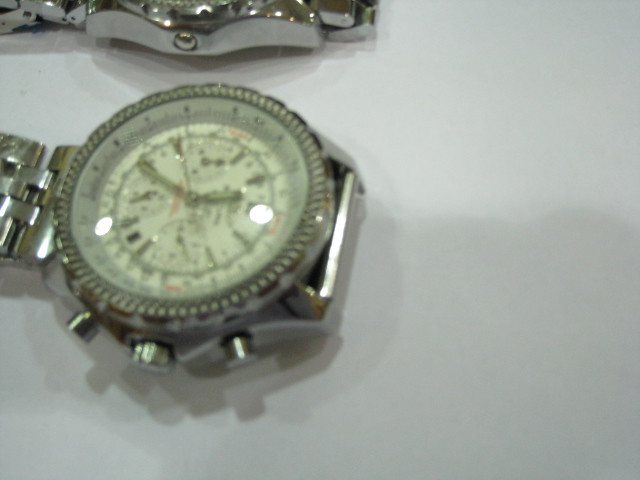A meticulously arranged image showcases two wristwatches against a pristine white background. The focal point of the composition is on the lower right side where one watch is prominently displayed. This watch, primarily detailed with silver hands and sleek white features, has a minimalist appeal with dashes marking the hours instead of numbers. A hint of red text is discernible on its face, though legibility is compromised upon closer inspection. The bracelet of this watch is crafted from polished metal, adding an element of sophistication. On the top left side of the image, a sliver of a second watch peeks into the frame, hinting at its presence with just enough detail to suggest a similar metal band. The overall hue of the image leans towards a yellowish tint, further accentuating the metallic elements of the watches. Despite efforts to zoom in for more detailed scrutiny, the brand names remain elusive, adding a layer of mystery to these elegant timepieces.